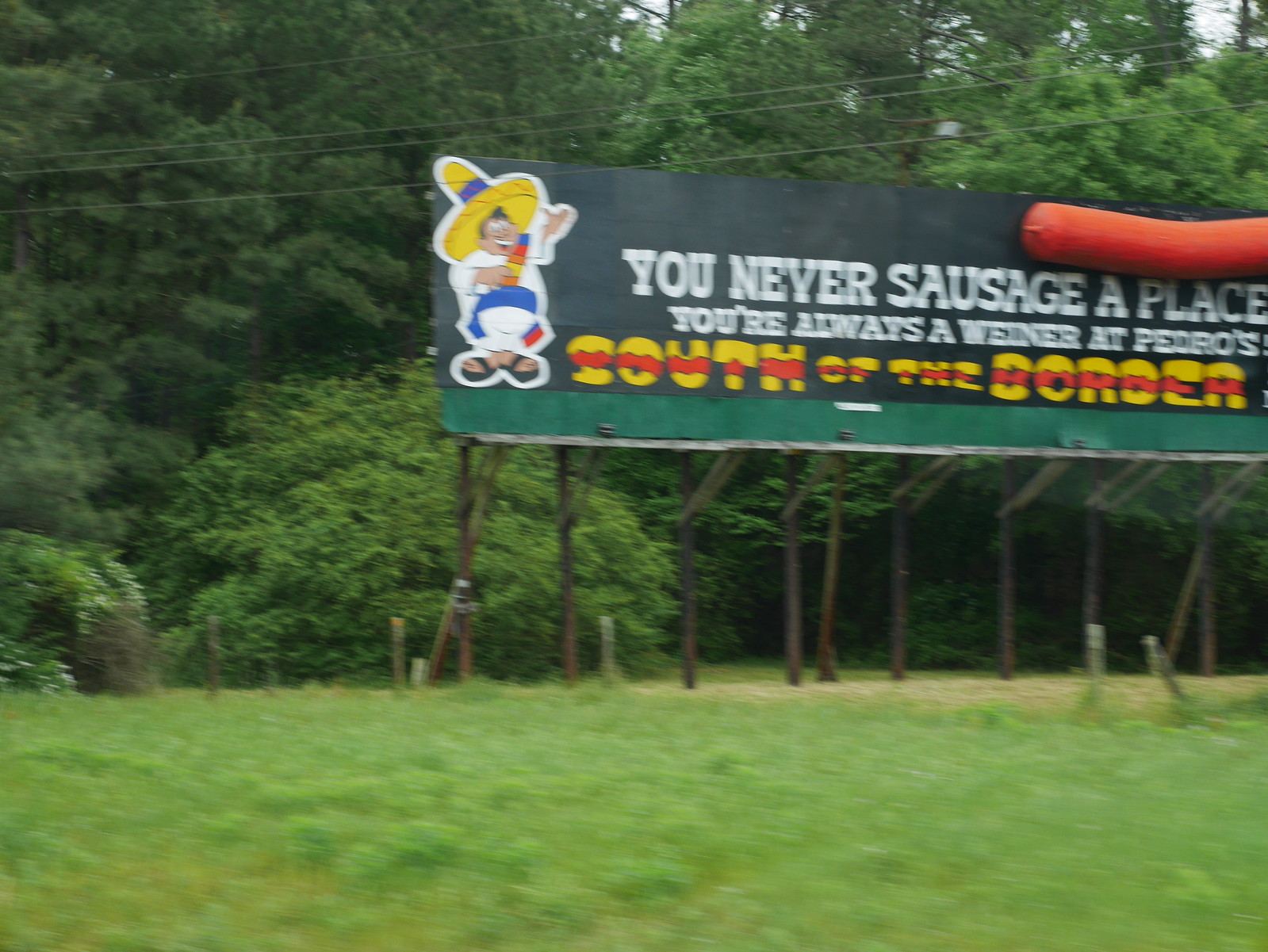The image showcases a billboard advertising the business South of the Border. The bottom section of the sign prominently features the South of the Border name in vibrant bubble letters, each character painted yellow with a red stripe running through the middle. To the left of the text, a whimsical cartoon character of a man wearing a sombrero is depicted, appearing to hold a bottle of hot sauce. Above the South of the Border logo, bold white letters spell out the playful phrase, "You never sausage a place." Directly beneath this line, smaller text humorously states, "You're always a wiener at Pedro's." Enhancing the billboard's three-dimensional appeal, a large, protruding sausage, which closely resembles a hot dog, extends slightly from the otherwise flat surface of the billboard, adding an eye-catching element to the advertisement.